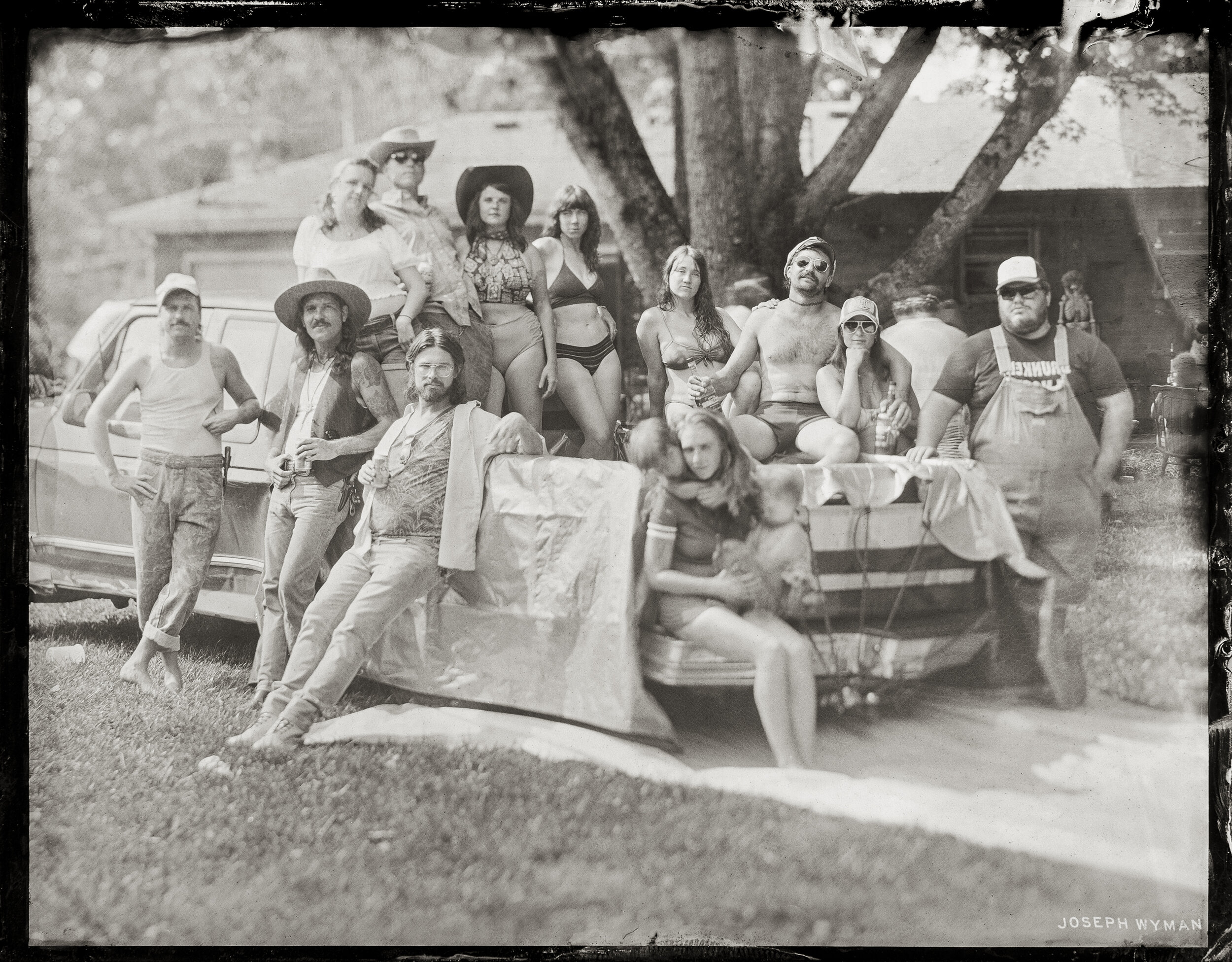This black and white photograph, with a thin black border, captures a nostalgic scene from what appears to be the 1970s or 1980s. A large group of people, exuding a carefree, hippie vibe, are either gathered around or lounging in the bed of a sizable old pickup truck parked on grass. The truck bed has been converted into a makeshift pool with a large plastic sheet and tarp, suggesting a playful summertime water slide setup extending from the rear.

Many of the individuals, dressed in bikinis, sleeveless shirts, or simply shirtless, indicate a hot summer day. They sport dark sunglasses and some wear cowboy hats, highlighting the eclectic styles of the era. The diverse group includes men and women, with some women holding children on the truck's bumper, adding a familial and communal touch to the scene. Their relaxed postures and the presence of drinks like beer underscore the festive atmosphere.

In the backdrop, a single-story house is partially visible, along with a towering tree providing ample shade. The setting is a mix of natural elements and human activity, with additional people seen mingling near the house. This highly detailed image effectively encapsulates the spontaneous joy and communal spirit of an outdoor summer gathering from a bygone era.